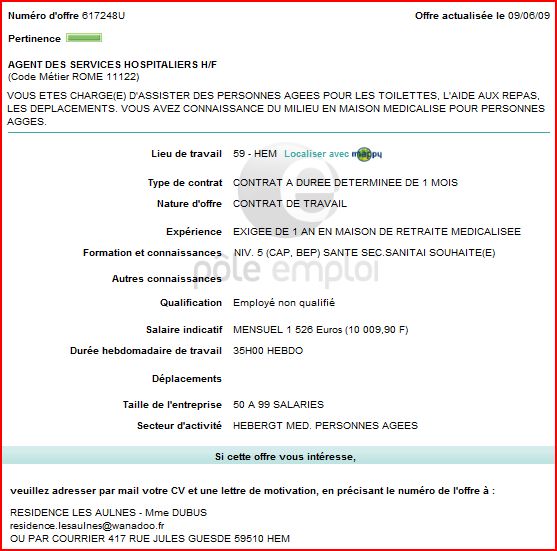This vertical rectangular image showcases a document with a distinct red border and primarily black text, featuring a structured format where various categories are followed by corresponding entries. The document is not in English, seemingly in French, and includes several highlighted segments in turquoise. At the top, a specific document number "Numero Dofra 617248U" is visible alongside a date "090609", and a heading labeled "Pertinence" accompanied by a green bar. Below this, there is a central section packed with extensive text written in capital letters, denoting information such as "Experience". Highlighting continues with a prominent turquoise line running horizontally. Further down, specific details include addresses and an email "residence.lesaulnes@wannado.fr," indicating potentially crucial contact or location information.